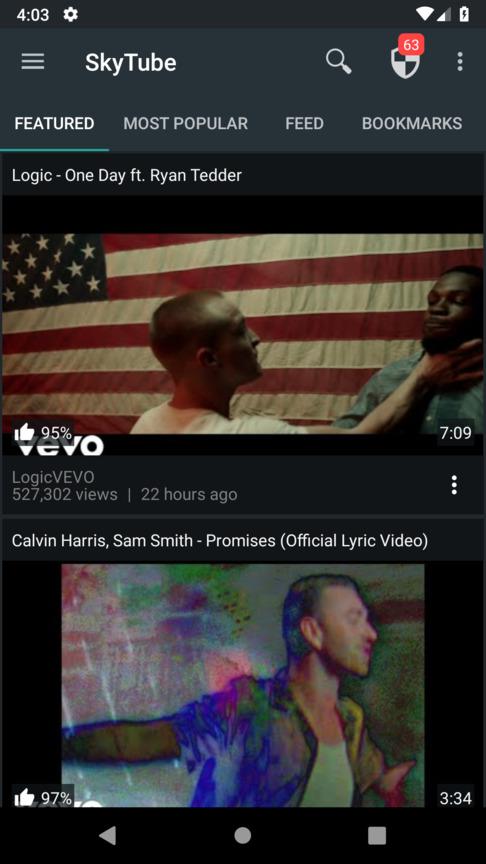The image captures the screen of a cell phone with a black background, prominently showcasing a couple of photos and various user interface elements. At the top of the screen, the time is displayed as 4:03, along with icons for settings (represented by gears), cellular connection, and a near-empty battery indicator. Directly below these icons is a search box with the term "SkyTube" inside it. Centered within the screen is a shield icon with a red "63" superimposed over it.

The interface is divided into four tabs horizontally across the page: "Featured," "Most Popular," "Feed," and "Bookmarks." The "Featured" tab is highlighted and underlined, indicating it is the currently active section. 

Below the tabs, on the left side of the screen, is the text "Logic One Day Featuring Ryan Tedder." This is followed by the first photo, which serves as a thumbnail. The image has the American flag as the background and features an African American man in a white t-shirt gripping the throat of another African American man in a green shirt. A thumbs-up icon with a "95%" approval rating appears next to the image, and the number "709" is displayed in the bottom right corner. Below this photo, the text reads "Vivo" and further states "Logic Vivo 527,302 views 22 hours ago."

Next, there is a description of another video titled "Calvin Harris Sam Smith - Promises (Official Lyric Video)." Accompanying this description is a profile image of a man looking to the right, with his arms spread wide, wearing a t-shirt layered under a long-sleeve shirt. Similar to the previous image, a thumbs-up icon with a "97% approval rating" is shown, along with the number "334" in the bottom right corner.